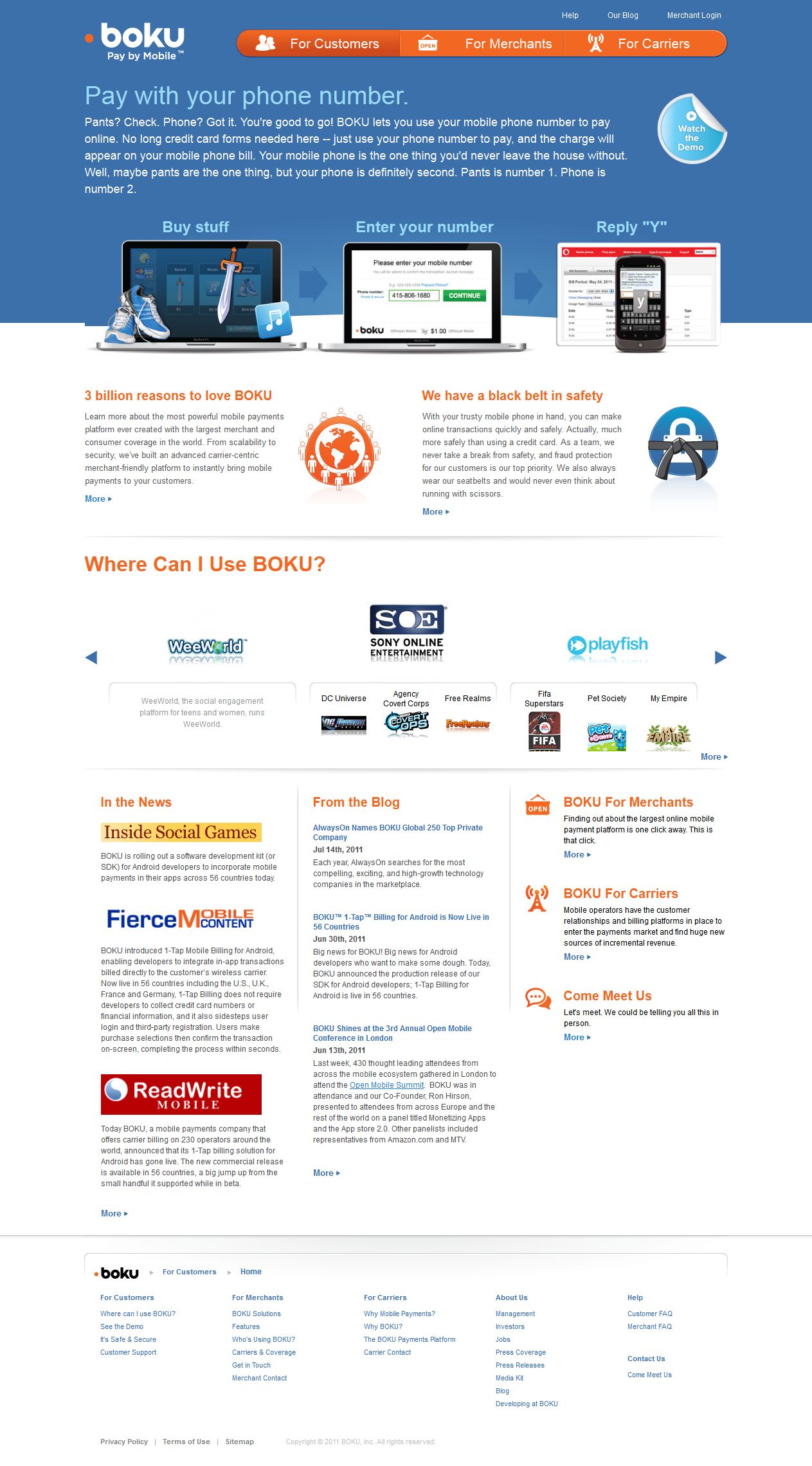Screenshot of the Boku Homepage in Landscape Mode

The screenshot showcases a large, detailed homepage of Boku, a mobile payment service. Dominating the upper left corner is a bold blue section featuring the text "Boku: Pay by Mobile." In the upper right corner, options for "Help," "Our Blog," and "Merchant Login" are easily accessible. 

Centrally located at the top, three prominent orange buttons are labeled for different user categories: "For Customers," "For Merchants," and "For Carriers." Just below this navigation bar, a catchy slogan reads, "Pay with your phone number. Pants? Check. Phone? Got it. You're good to go." This is followed by an explanation of how Boku works, highlighting the ease of using your mobile phone number to make online payments without lengthy credit card forms. The charges appear directly on your mobile phone bill.

A playful note emphasizes the importance of one's mobile phone, ranking it just behind pants as an essential item when leaving the house. To the right, an interactive circle element invites users to "Watch the Demo."

Further down the page, three illustrative images are displayed in a row. The first image shows a laptop alongside sneakers, a sword, and music icons with the caption "Buy Stuff." The second image instructs users to "Enter your number and reply Y." Finally, the third image champions Boku’s security with the statement "Three billion reasons to love Boku. We have a black belt in safety."

The page continues with sections that answer "Where can I use Boku?" and provide additional information "In the News," "From the Blog," "Boku for Merchants," and "For Carriers." An invitation to "Come Meet Us" rounds out the detailed and user-friendly overview of Boku's innovative mobile payment service.